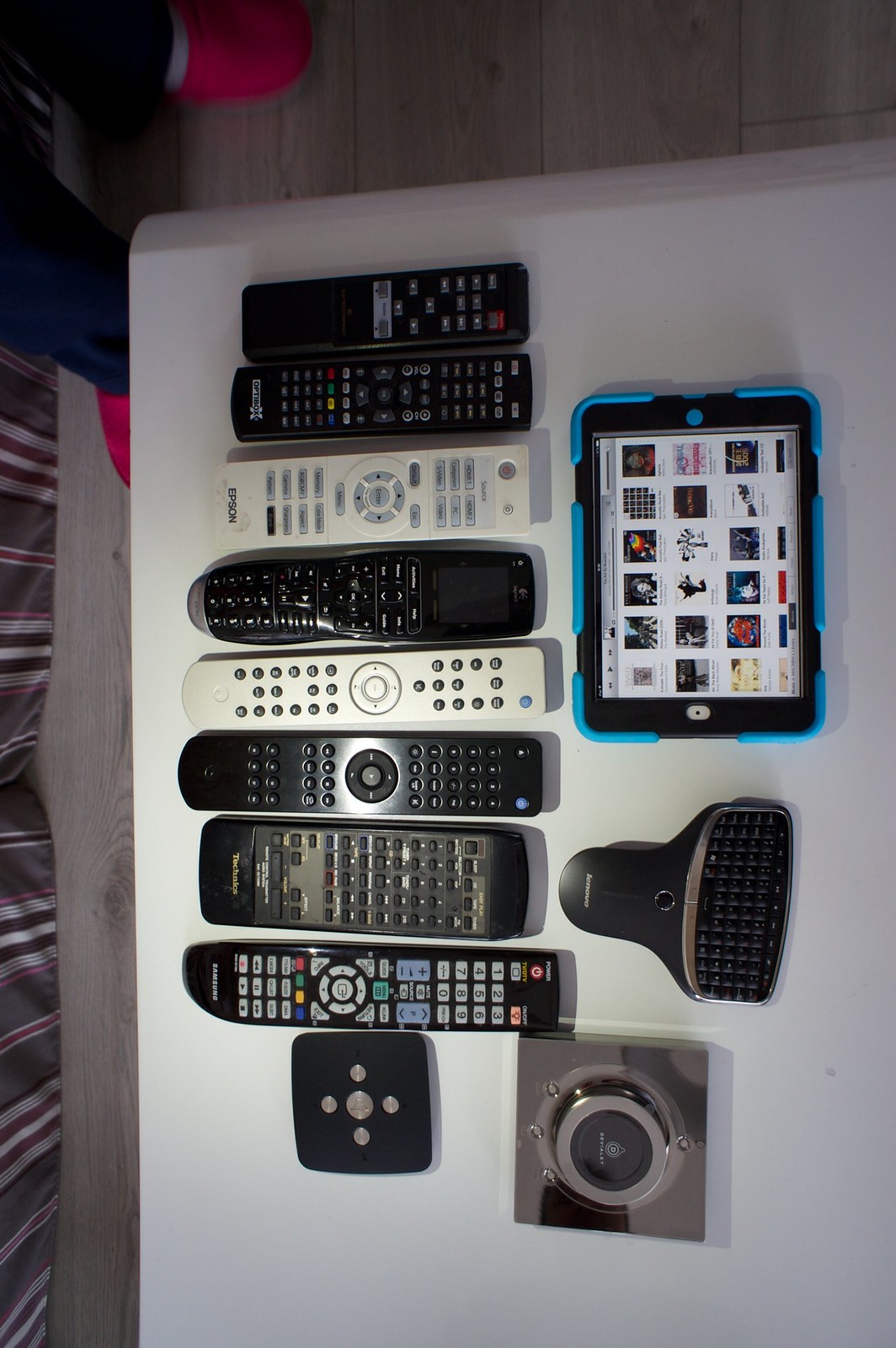In this overhead photograph, a white tabletop is cluttered with various electronic devices, all set against a backdrop that includes a wooden floor and hints of curtains on the left edge. Dominating the table are eight remote controls, six black and two white, each designed for different TVs or electronic devices with varying button layouts. Near the remotes is a tablet encased in a blue rubber safety cover, its screen displaying numerous small, indistinct images. Adjacent to the tablet lies a Bluetooth keyboard and a sleek, silver trackpad. In the background below the table, the wooden floor is visible, as are the feet of a person in red shoes.